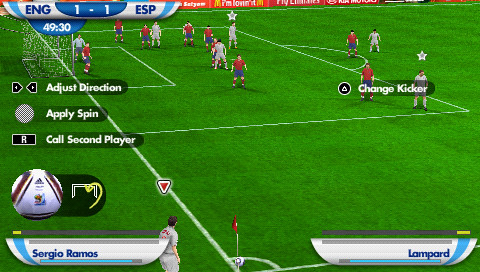A detailed screenshot of a soccer video game in progress, featuring a simulated scoreboard prominently displayed in the top left corner. The scoreboard indicates the match is between England (ENG) and Spain (ESP), with a current tied score of 1-1 highlighted in a blue section. Directly beneath the scoreboard, the game timer shows 49:30 minutes elapsed. Below the timer, text displays additional match details.

Further down the screen, there's a prominent rectangle with the letter 'R' in the middle, accompanied by a prompt that reads "Call Second Player." At the very bottom, player names are displayed on banners: Sergio Ramos on the left and Lampard on the right, indicating the players currently involved in the action.